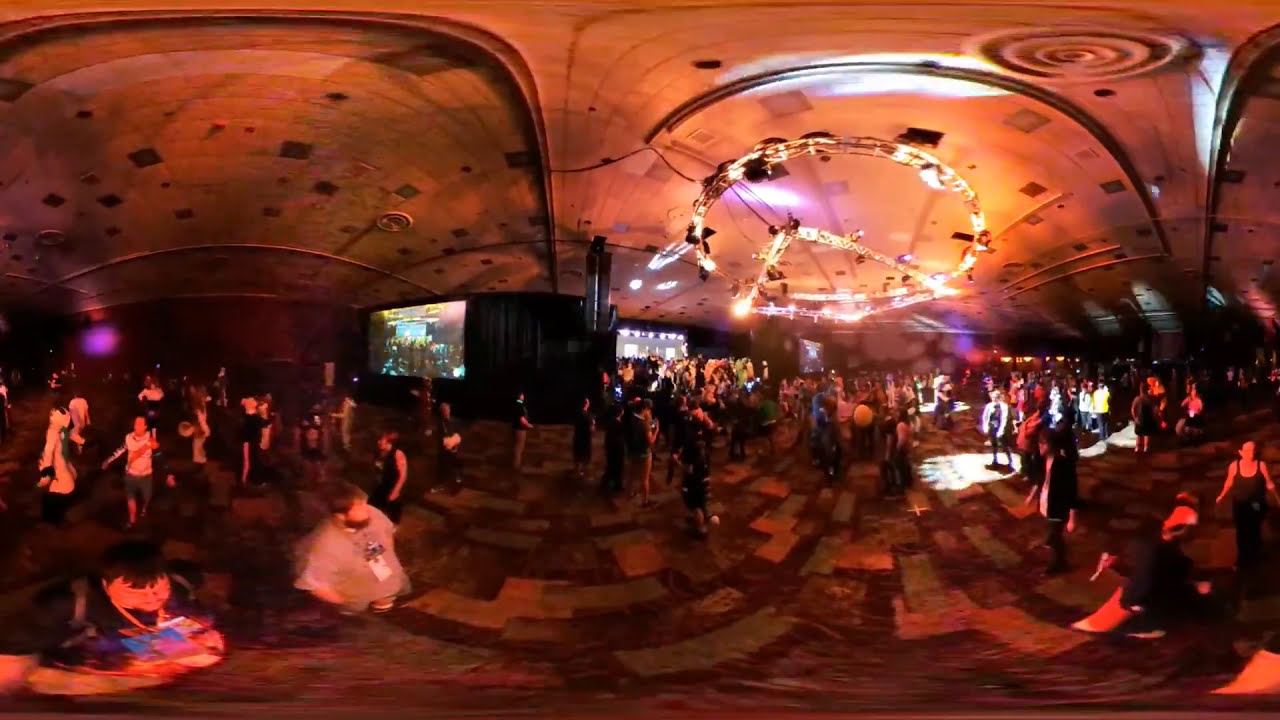The image portrays a bustling scene inside a club or convention, captured through a fisheye lens that creates a 360-degree view. The ambiance is awash with a mix of red, pink, blue, purple, orange, brown, black, white, and yellow hues, giving it a lively, vibrant atmosphere. Several people, potentially attending a celebration or performance, are scattered across the scene, engaging and interacting with each other. Large screens are visible in the background, enhancing the energetic setting. Overhead and side lighting, including distinct spotlights on the right and left, create a cool yet somewhat dim vibe. The floor appears to be a mix of tiles or carpet, possibly enhanced by special effects. The layout is rather chaotic, with objects and individuals dispersed throughout the image. Notably, there is no visible text anywhere in the picture.